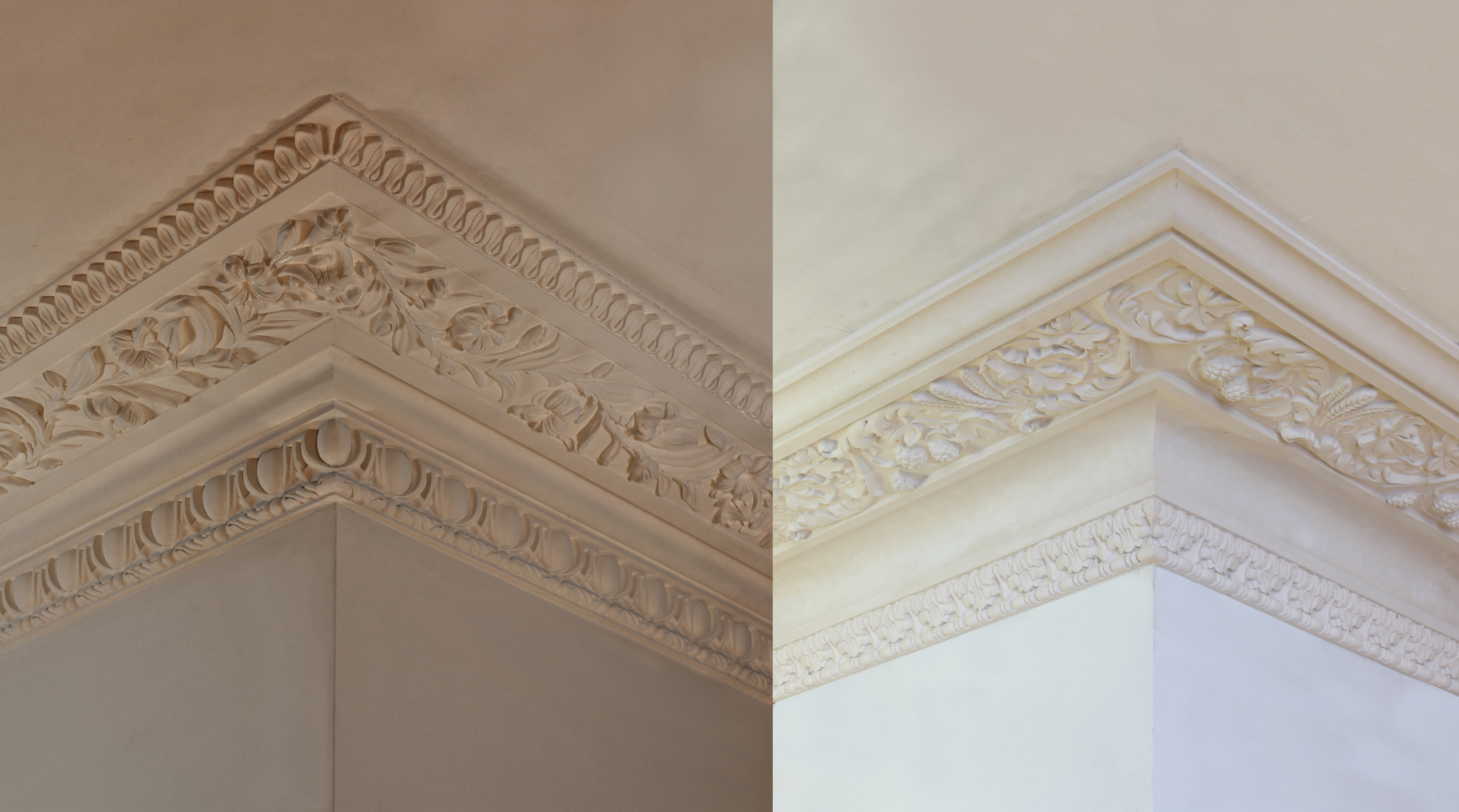This image shows a split view of two sections of a wall meeting the ceiling, both adorned with intricate plaster embroidery. The wall's base color is beige, and the top edge is decorated with detailed fresco-like plaster work. On the left side, the wall appears darker due to lower lighting and looks beige-pinkish, highlighting a more intricate S-pattern bordering with flower and leaf designs. The matching lower embroidery contains a circular piece nestled within a U-shaped design. In contrast, the right side of the image is better illuminated, revealing a primarily white wall with beige accents specifically at the embroidered sections. Here, the border design differs, featuring a simpler pattern with multiple circular shapes and other details substituted in the lower embroidery section. The division clearly shows both the differences in the plaster patterns and the effect of lighting on the wall colors.